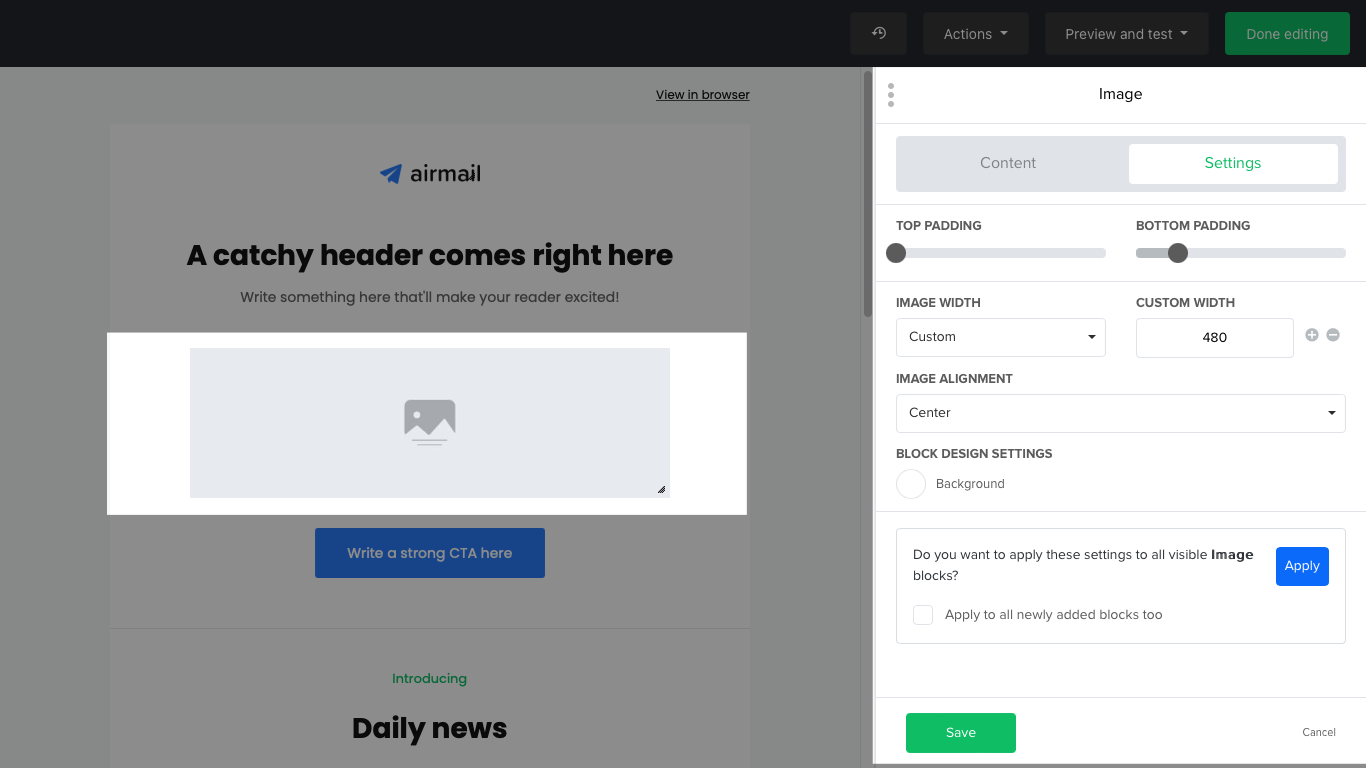This screenshot captures the Airmail website interface during the editing phase. Dominated by the Airmail logo prominently displayed towards the top center, it features a "View in Browser" link situated near the top, slightly right of center. A black navigation bar at the very top contains several functional icons, including a clock, a reverse action button, a preview, and a test button, alongside a green "Done Editing" button.

The right-hand side of the page is dedicated to an editing panel labeled "Settings." Here, options are available for adjusting top and bottom padding, as well as image width — set to a custom value of 480 pixels. Users can easily modify this width using adjacent plus and minus buttons. The interface also allows for image alignment configuration, currently centered, and includes block design settings, with an option to set a background.

Beneath these controls, a thin gray box prompts the user with the question, "Do you want to apply these settings to all visible image blocks?" with an accompanying blue button to apply the changes uniformly. Additionally, there is a checkbox to enable these settings for all newly added blocks. The bottom of this interface features a green "Save" button on the left and a cancel button on the bottom right, offering a clear way to finalize or discard changes.